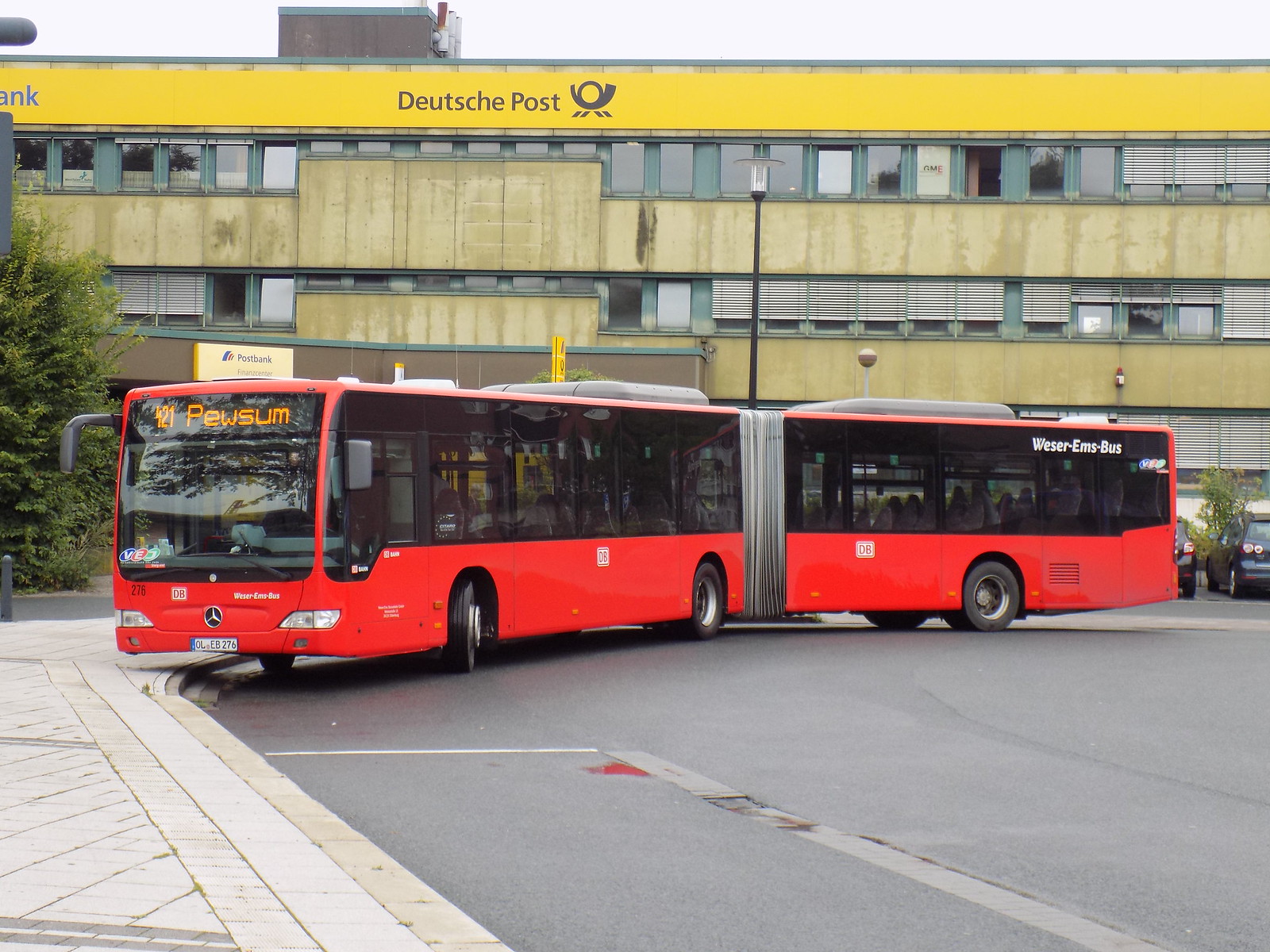This outdoor scene features a striking long red double bus rounding a curb, prominently marked with the number 421 and the destination "PEWSUM" in capital orange letters on the front. The bus, separated into two connected sections, has high, flat, clear windows. On its rear, the word "BUS" is visible in white letters, starting with a discernible "W." Adjacent to the bus is a light cement brick sidewalk.

In the background, an imposing industrial building stands out with its top level painted yellow, displaying the name "DEUTSCHE POST" and a black circular logo. The building, adorned with rows of large windows, some fitted with blinds, has green-painted areas surrounding the windows. The sky above is overcast, casting a gray hue over the entire scene.